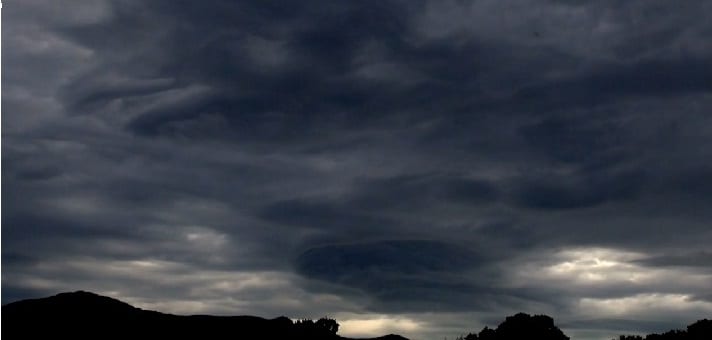The image captures a dramatic and very stormy sky, dominated by thick, dark clouds in various shades of gray and black, with patches of white and light gray scattered throughout, creating a moody and tumultuous atmosphere. The cloud formations have an almost smudgy, oil painting-like texture, and thin enough in places to reveal subtle hints of sunlight on their edges, suggesting either sunrise or sunset. Below this menacing sky lies a silhouette of a hilly landscape, with blackened hilltops and sparse grassy areas visible. On the left side, there is a prominent hill, with a smaller mound in the center, while the bottom right corner reveals a cluster of grass and another small hill. The image is devoid of visible wildlife, adding to the stark, almost eerie quality of the scene.